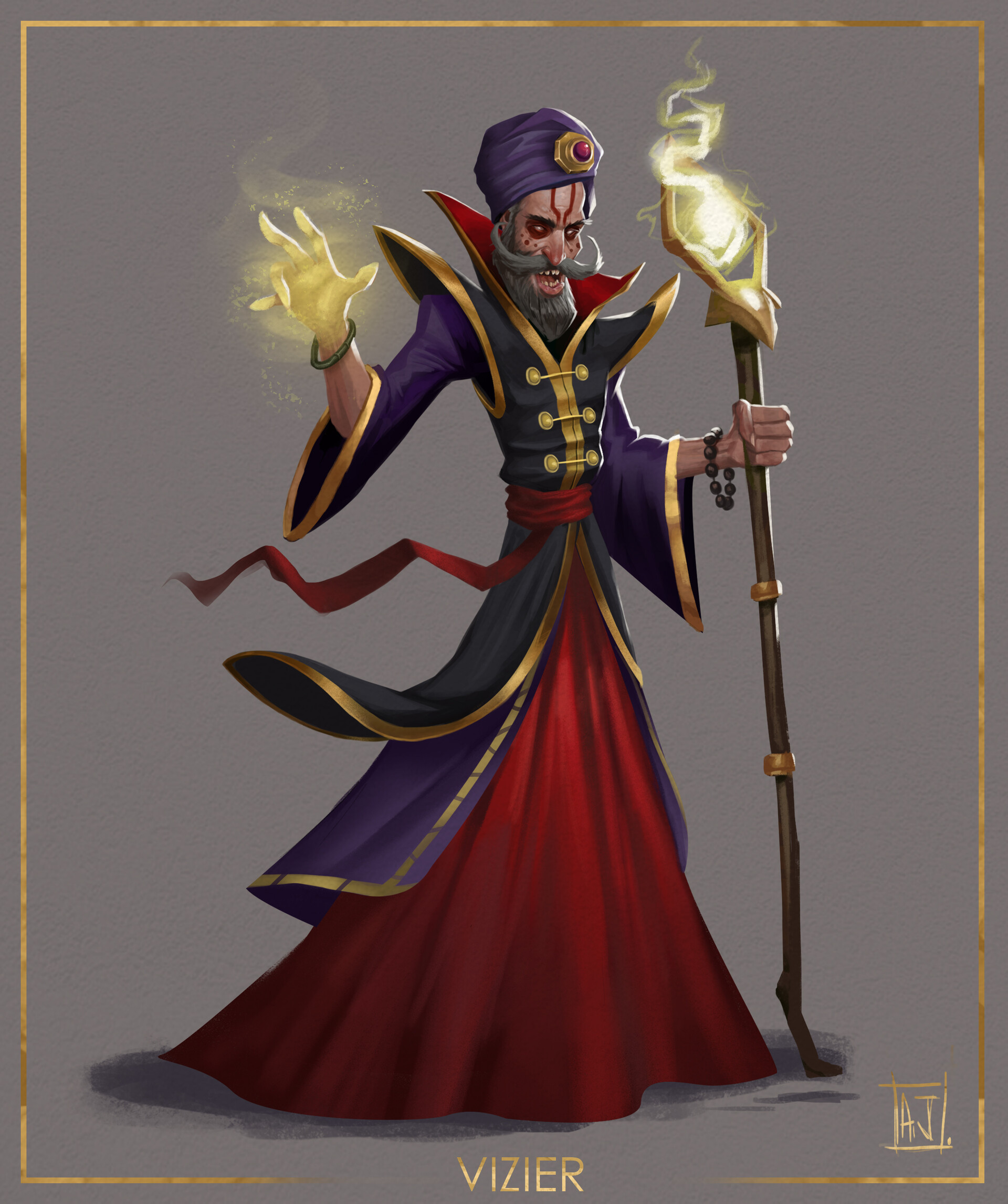This detailed illustration depicts a wizard-like character reminiscent of a villain from Aladdin. At the bottom of the image, the title "Vizier" is displayed in gold text, accentuated by a gold square border around the image. A logo featuring the initials "A-J" in gold is positioned at the bottom right.

The wizard's attire is elaborate, featuring a dark blue and gold cloak with red interior, complemented by a red skirt-like garment and a purple tunic. He wears a purple turban adorned with a gold pendant, centering a ruby. His wrists are decorated with bracelets – a beaded one on the left and a plain black one on the right.

In his right hand, the wizard firmly grasps a staff topped with a diamond-shaped gold ornament emitting gold-colored smoke. His left hand is raised, conjuring a spell that manifests as golden light. Notably, there appears to be blood trickling from his eyes, adding a menacing touch to his mystical presence.